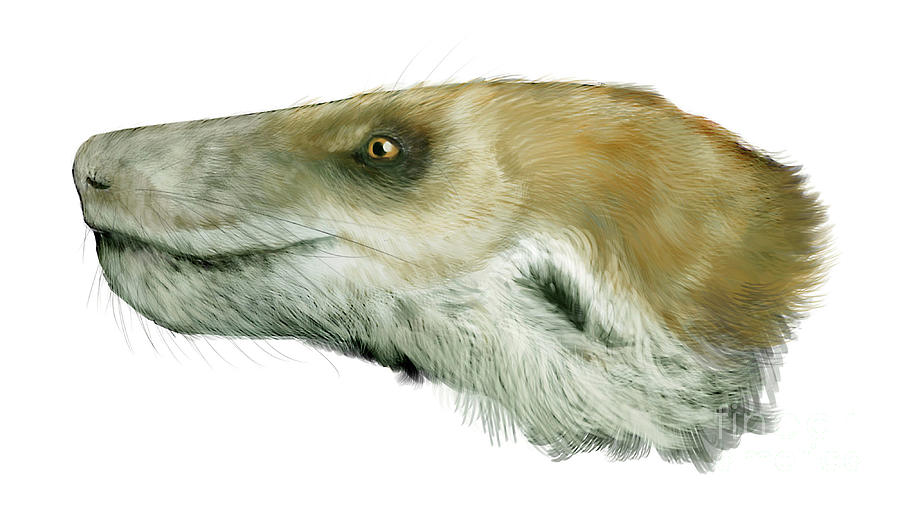This is a meticulously detailed photographic-style image of a mammal's head, resembling a prehistoric creature, presented on a solid white background. The image dimensions are rectangular, with the top and bottom sides being twice as long as the left and right sides. The animal's head faces left, showing its unique blend of fur colors and intricate features. The head is depicted from the snout to the beginning of the neck, with the mouth closed and tapered nose, and extends slightly beyond the midpoint to the right of the image.

The creature boasts a complex coloration pattern: tan gold fur covers the back of its head and neck, transitioning to darker brown fur towards the edge of the image. The front of the face features grayish and whitish fur, with long black whiskers sprouting from the sides of the nose and chin. The eye, positioned slightly more than halfway to the left, is orange with a black pupil, surrounded by light and dark brown fur, creating a striking contrast. Below the eye and around the mouth, patches of gray, black, and white fur intermingle. A presumed ear opening is marked by a black spot on the side of its head.

Overall, the mammal displays a blend of light and dark tones throughout its fur, with the darker hues concentrated towards the back end of the head, giving it a richly detailed and lifelike appearance. There is no text in the image, keeping the focus solely on the creature's striking visage.